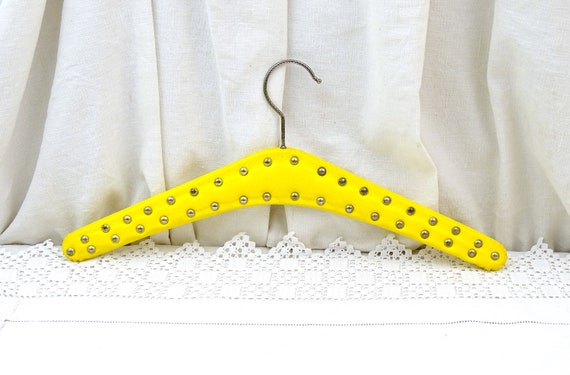The image shows a highly detailed and vibrant yellow coat hanger, resembling the shape of a boomerang. The hanger is covered in yellow felt material that extends from the base of the hook to each end. This material is adorned with small, round silver rivets that line both edges of the hanger. The top of the hanger features a sleek, silver metal hook. The hanger is propped against a backdrop that includes a white bed skirt and a bright white lace or doily-like fabric on the floor, providing a textured and decorative contrast. In the background, there is a slightly brownish tint on the left side of the curtain, adding depth to the scene.